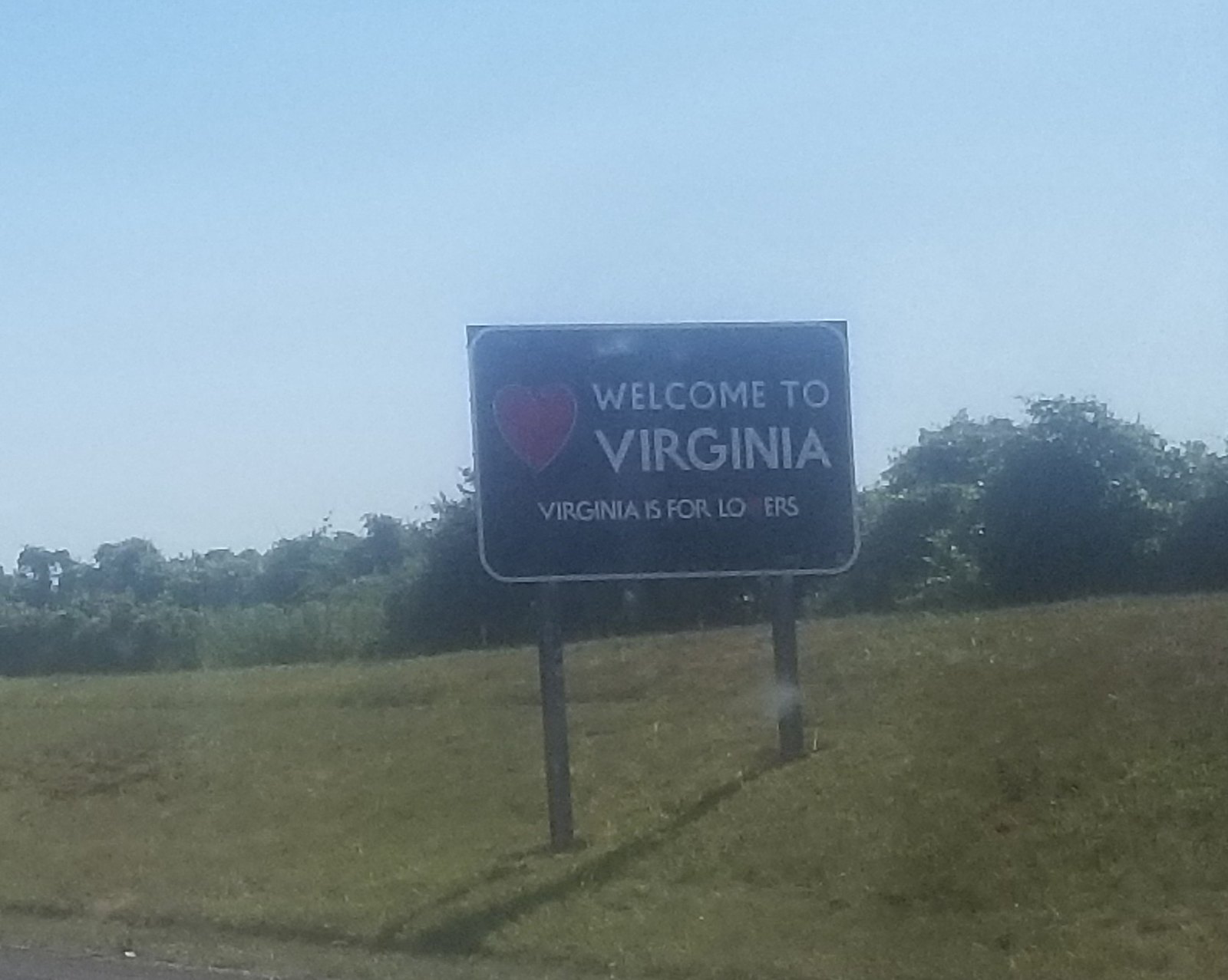A roadside sign welcomes drivers to Virginia, featuring the slogan "Virginia is for lovers" — though the letter "v" is missing, leaving a noticeable gap in the text. The sign, displaying a large red heart, appears worn and weathered, particularly evident above the "Welcome" text and around the heart. Captured from a moving car, the photo shows reflections on the window, slightly obscuring the view. Below the sign, a patch of grass leads to a thicket of trees and brush, framing the sign in a natural roadside setting.